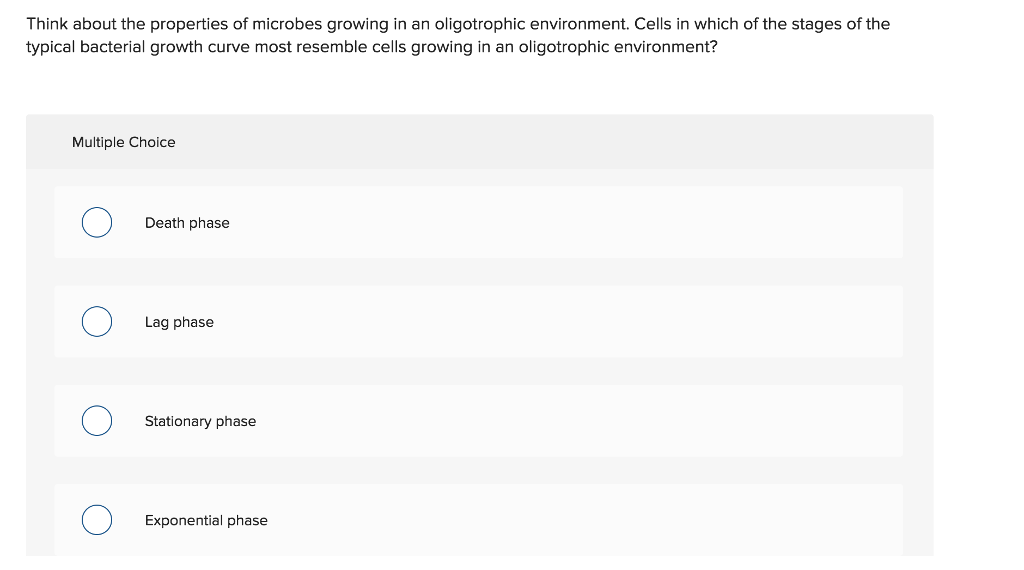"An image snippet from a test showcases a single multiple-choice question accompanied by four possible answers. The screenshot captures a clean interface with a white background at the top, displaying a question in dark gray font: 'Think about the properties of microbes growing in an oligotrophic environment. Cells in which of the stages of the typical bacterial growth curve most resemble cells growing in an oligotrophic environment?' Below, a light gray rectangle introduces the multiple-choice section on the left. Each possible answer is enclosed in its own rectangle, in the same gray font. They are as follows: 'Death phase,' featuring an adjacent white circle for selection; 'Lag phase'; 'Stationary phase'; and 'Exponential phase,' each with a corresponding white circle beside them for the user to click and indicate their selection."